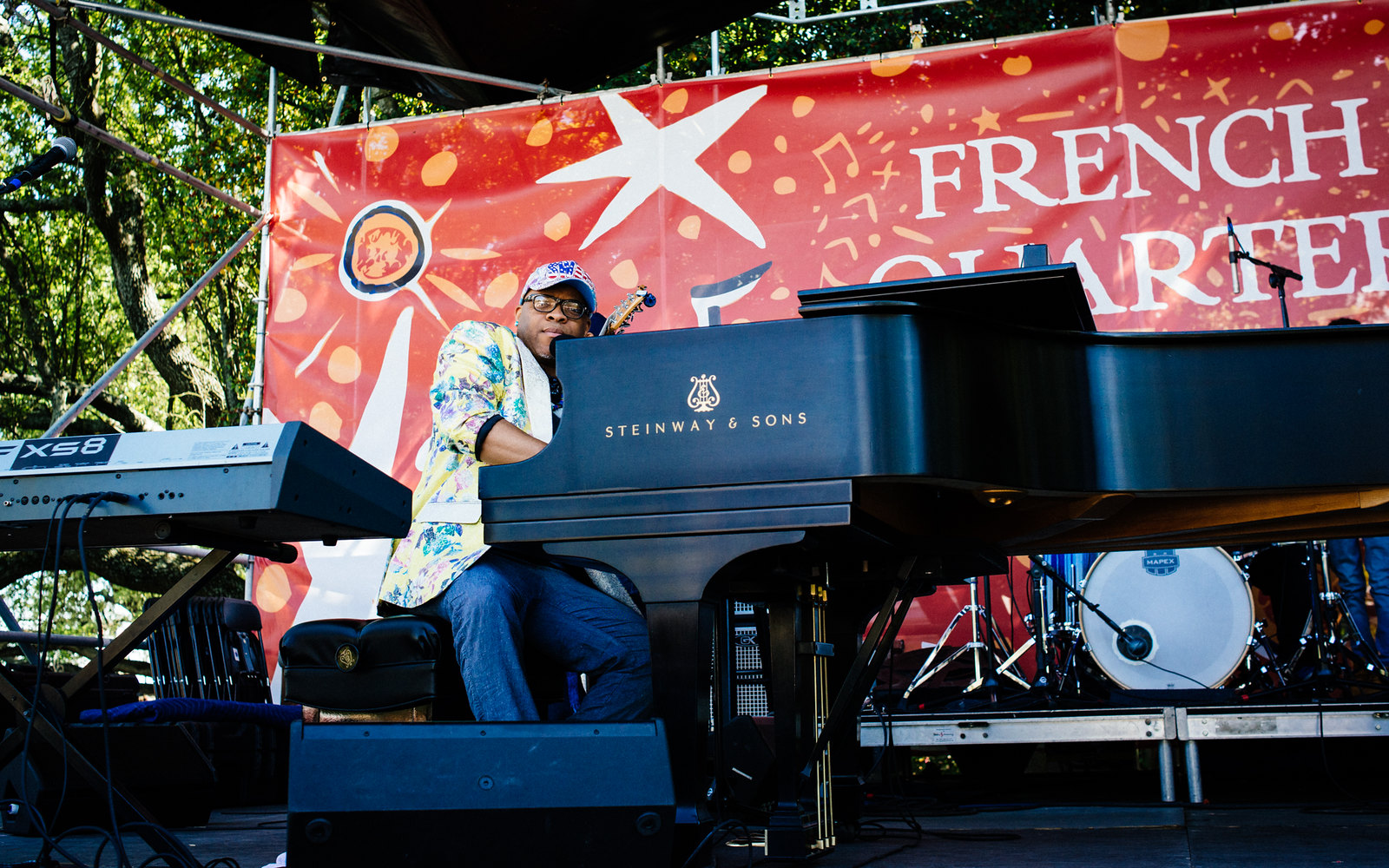In this detailed close-up photograph of an outdoor concert event, the focus is on a black pianist seated at a grand Steinway and Sons piano, its brand name elegantly showcased in gold text on the side, alongside the iconic harp logo. The pianist is distinguishable by his thick black glasses, white hat, and rolled-up sleeves of a white jacket, complemented by blue jeans. Surrounding him is a vibrant scene: a red banner adorned with orange dots, circles, hearts, stars, musical notes, and dashes stretches across the stage's background. The white text on this banner reads "French Quarter," suggesting the event's location within the lively French Quarter. Partially visible next to the piano is a drum set tucked under the stage's platform. The photograph also captures elements of the stage structure, including the metal supports of the overhead cover and glimpses of green trees beyond the tented area, framing this energetic moment in an atmospheric outdoor performance.